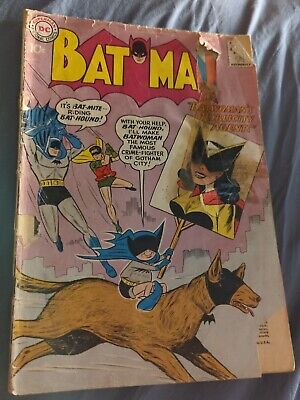This image depicts a highly worn and visibly aged Batman comic book, likely from around 50 years ago. The cover features the classic Batman logo in white font on a red background, partially obscured by damage and tearing, particularly on the upper right corner where some pieces are missing, possibly including the price. The DC logo is set in a circle at the upper left corner. Central to the image are Batman and Robin, clad in their traditional blue, yellow, red, and green costumes, depicted mid-action as they swing downwards. They appear alongside Bat-Mite, a child-sized character in a miniature Batman costume, riding Bat-Hound, a brown dog with a black mask and a bat collar. Bat-Mite holds a sign representing a vintage Batwoman, adorned in a yellow top, black mask, and red cape, proclaiming her as "Batwoman's Publicity Agent." Behind this lively scene is a faded cityscape. The cover also shows signs of water damage, especially along the right side, adding to its distressed appearance.